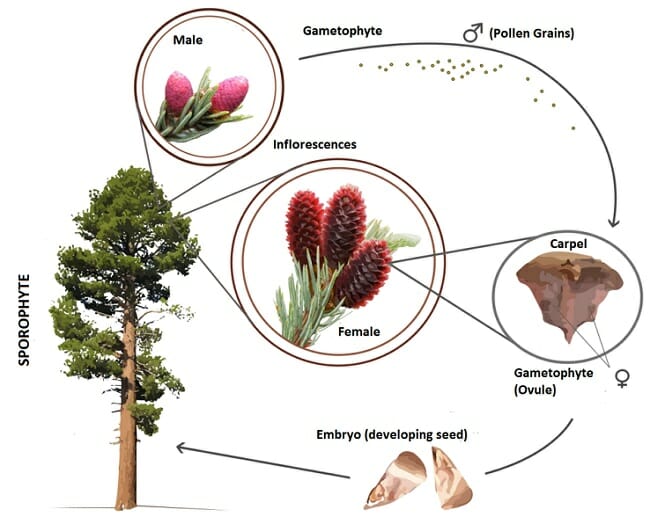The image is a detailed lifecycle diagram of what appears to be an evergreen tree, presented against a white background with no boundaries. On the left side of the image, a tree with a brown trunk and green leaves is labeled "sporophyte" in vertical black letters. Moving clockwise, there's a magnified section of the tree showing a male gametophyte within two concentric dark brown circles. It depicts small green leaves and two pink, egg-shaped components, labeled "male" with a male symbol and "pollen grains."

An arrow with green dots beneath it curves towards the center of the image, pointing to a red spiky structure encircled twice with dark brown rings. This part is labeled "female" and "gametophyte," with a female symbol and the term "ovule." V-shaped lines connect this image to another magnified part labeled "carpel" (C-A-R-P-E-L) containing an irregular brown shape.

A curved line from the carpel leads to two "embryo" images at the bottom of the chart, labeled as developing seeds in dark brown, white, and light brown colors, resembling long triangles with rounded ends. From these embryos, a straight black arrow points back to the tree, completing the lifecycle. Throughout the diagram, different components are visually linked to show the progression from gametophytes to sporophytes, emphasizing the cyclical nature of the tree's reproduction process.